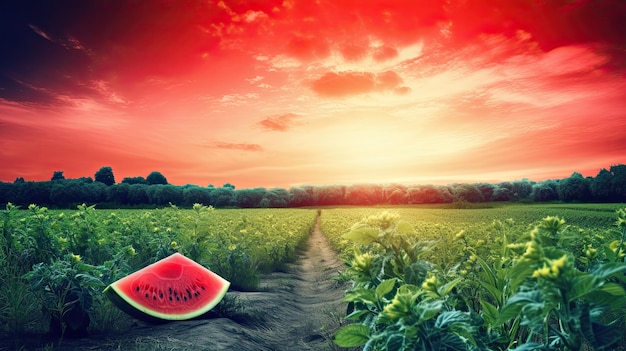The photograph captures a surreal, vividly enhanced sunset with a bright reddish-yellow sky, transitioning from a yellow center to a deep red at the top. Beneath this striking sky, a thick line of dark green trees stretches across the horizon. In the foreground, rows of green-leafed crops, adorned with sporadic yellow flowers, extend orderly across the image. A narrow, dirt pathway runs down the center, barely wide enough for a single person, guiding the eyes towards the bottom right where a conspicuously vibrant slice of watermelon rests on the soil. This watermelon wedge, with its deep red flesh, white rind, green skin, and scattered black seeds, stands out starkly as though photoshopped into the scene, adding an element of surrealism to an already vividly filtered farm landscape.